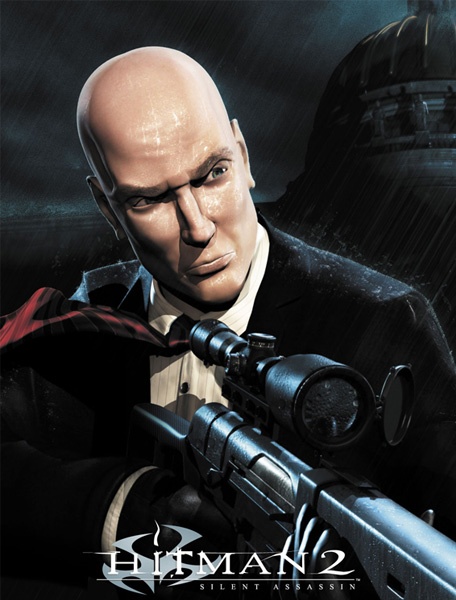The poster for the video game "Hitman 2: Silent Assassin" features a dramatic and intense scene. At its center stands a bald man with a serious expression, looking off to the right. He is immaculately dressed in a black suit, white shirt, and a red tie that is draped over his right shoulder. The man is holding a large black sniper rifle equipped with a prominent scope, ready to aim. The game's title, "Hitman 2," is displayed prominently at the bottom in large white letters, with "Silent Assassin" subtitled beneath it in smaller white letters. The background is dark and rainy, accentuated by streaks of light reflecting off the man's face and suit, emphasizing the intense atmosphere. A large, dark, dome-like structure reminiscent of a capitol building looms in the rainy backdrop, enhancing the ominous mood of the scene. This computer-generated image captures the essence of the game's stealth and precision.